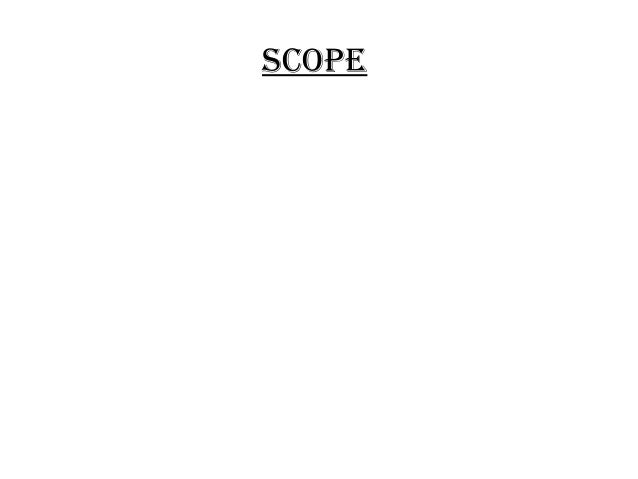The image features a stark plain white background with no borders. Dominating the upper center is the single word "SCOPE," rendered in small black, capitalized letters, each framed in white. Beneath the word, there is a black underline that accentuates the text. The font size is modest, with each letter measuring about half an inch or slightly less. The simplicity of the image is striking, with no other objects or elements present, creating a clean and empty space that draws attention solely to the underlined word "SCOPE," set against the vast white expanse, possibly suggesting an introductory slide of a presentation.